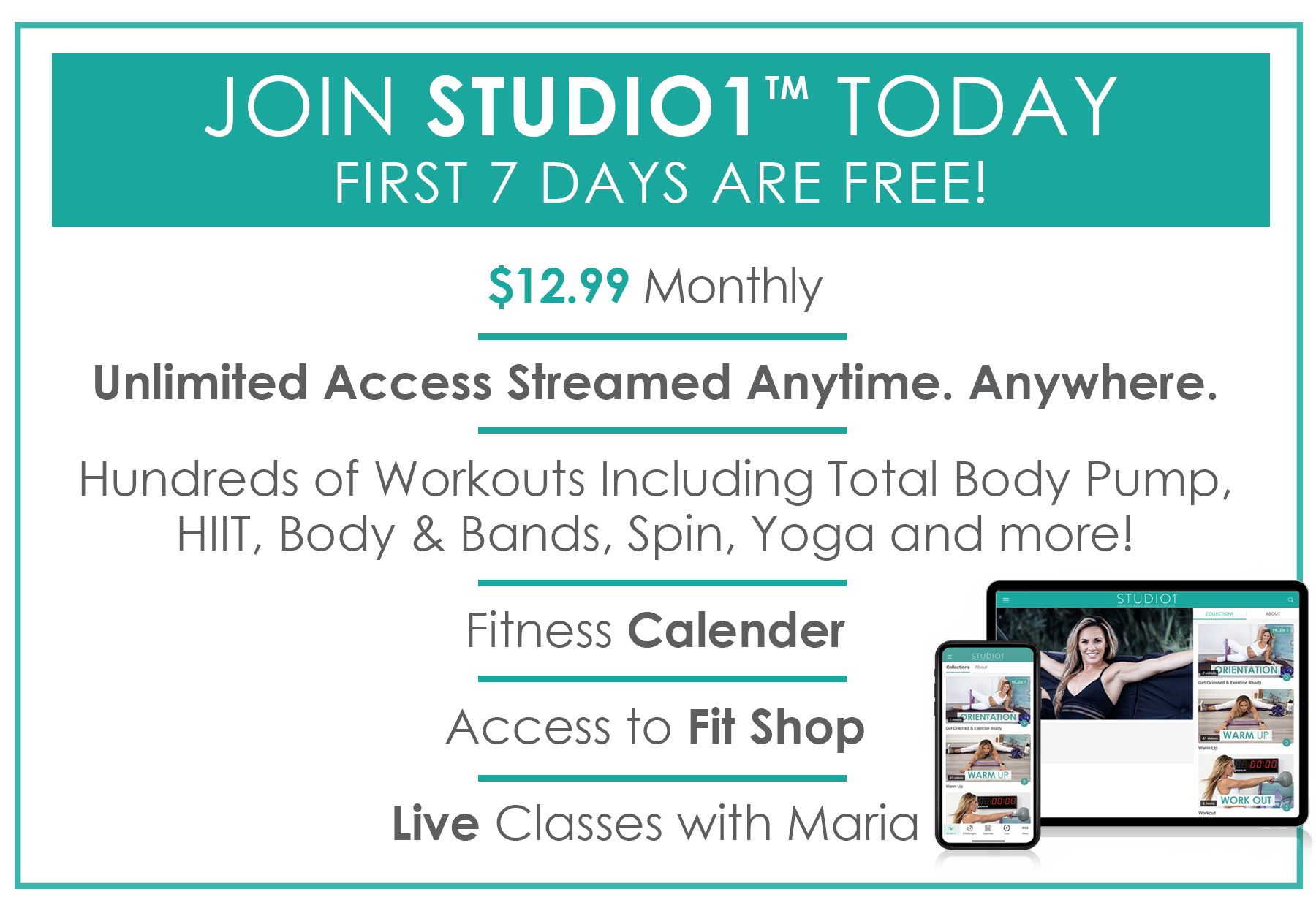**Join StudioOne™ Today: First Seven Days Free!**

The promotional image features a clean white background with a vibrant blue bar at the top, displaying the enticing offer to "Join StudioOne™ Today." The offer highlights that the first seven days are free. In bold blue text, "StudioOne" stands out, followed by the subscription cost of $12.99 monthly, which is underlined in blue.

Below this, the image details the benefits of joining StudioOne™. Subscribers get unlimited access to stream workouts anytime, anywhere. The platform boasts hundreds of workouts, including Total Body Pump, HIIT (High-Intensity Interval Training), Body and Band, Spin, Yoga, and more.

In black text, the image mentions a "Fitness Calendar," with "Calendar" emphasized in bold. It also grants access to the "Fit Shop," with "Fit Shop" also highlighted in bold. Green lines underneath "Fitness Calendar" and "Stream Anytime" add a pop of color to the design.

On the right side of the image, live classes with Maria are advertised, with "Live" in bold, suggesting the added benefit of real-time interaction. A visual of the website displayed on a tablet and a smartphone emphasizes the convenience and accessibility of the platform.

Overall, the image convincingly promotes StudioOne™ as a comprehensive fitness solution, readily available on various devices for a monthly fee of $12.99.